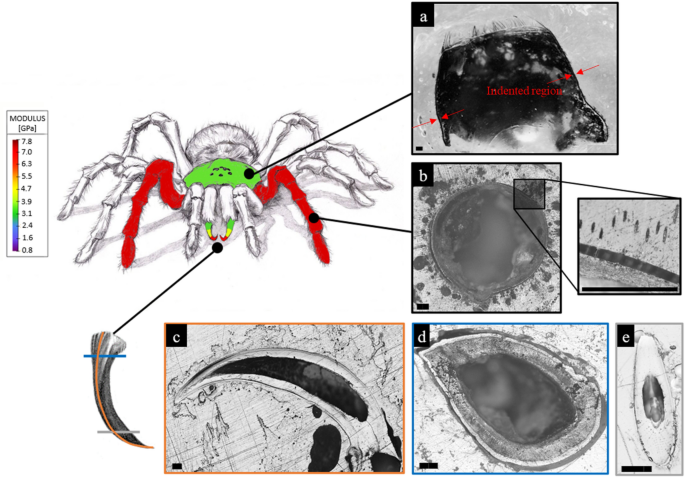This image is an intricate scientific diagram of a tarantula, featuring both an artistic line drawing and close-up microscopic views. The central figure is a black-and-white pen and ink illustration of the tarantula, facing towards the viewer, with specific parts highlighted in various colors. The upper body is colored in lime green, the front legs in red, and the fangs exhibit a gradient of green, yellow, and red. On the far left, there's a color-coded thermometer labeled "Modulus GPA," ranging from 7.8 to 0.8, with segments colored from red to dark blue, representing various stress limits on the tarantula's body. The right side and bottom of the image showcase six microscopic close-up photographs of different body parts of the tarantula, arranged and labeled A through E. Image A shows an indented head region, B displays part of a leg, C exhibits the fangs, and D features a world map-like structure and a black circular insert, the exact nature of which is unclear. E is a small circular diagram with a black insert, further drawing attention to the detailed anatomy of the tarantula. Overall, the image fuses artistic and scientific elements to provide a comprehensive understanding of the tarantula's anatomy.